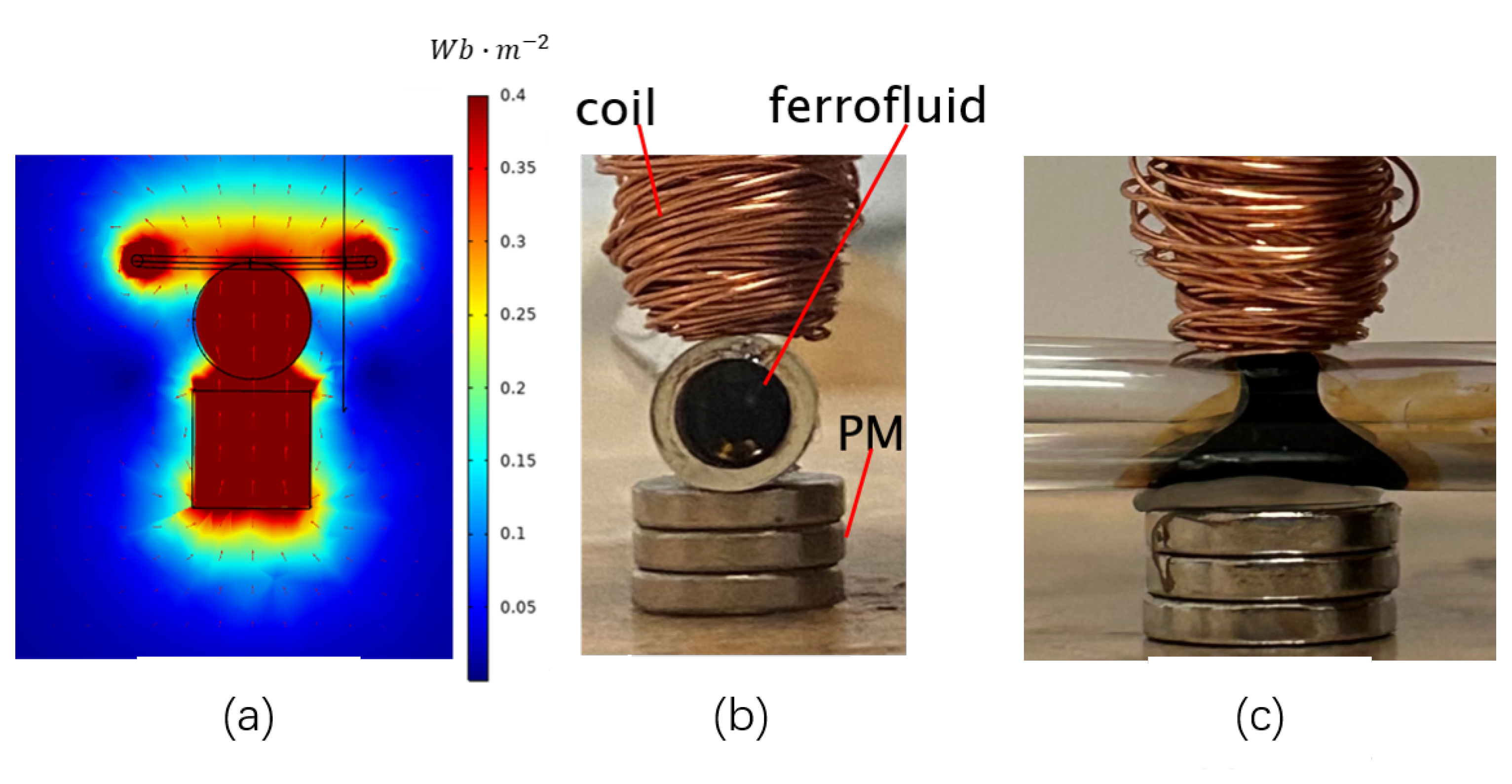This image presents a multi-part scientific illustration, consisting of three labeled sections (a, b, and c). 

In section **a**, on the left, there is a colorful thermographic image displaying various heat levels across an object. The background is predominantly blue, indicating cooler temperatures, while concentric bands of aqua, yellow, and red reveal areas of increasing heat. The diagram features a central circular area with two smaller round circles placed symmetrically around it. Below this central area lies a larger circle followed by a square at the base. Measurements and color-coded scales are adjacent to this section to quantify temperature variations.

Section **b**, positioned in the middle, showcases a realistic depiction of the object seen in section a. It consists of a stacked arrangement with three circular metal disks at the bottom. A metal tube labeled "ferrofluid" extends upwards from the disks, with an arrow pointing to its interior. At the top, a copper coil of wire, designated as "coil," is wrapped around the tube. Additionally, a label marked "PM" and connected by a red line points to the silver nuts or bolts resting on the metal disks.

Section **c**, on the right, provides a close-up side view of the arrangement displayed in section b. This image emphasizes the three metal disks at the bottom, the ferrofluid tube in the center, and the copper coil at the top from a different perspective.

Each section contributes to a comprehensive and detailed visual explanation of the scientific experiment or device being illustrated.